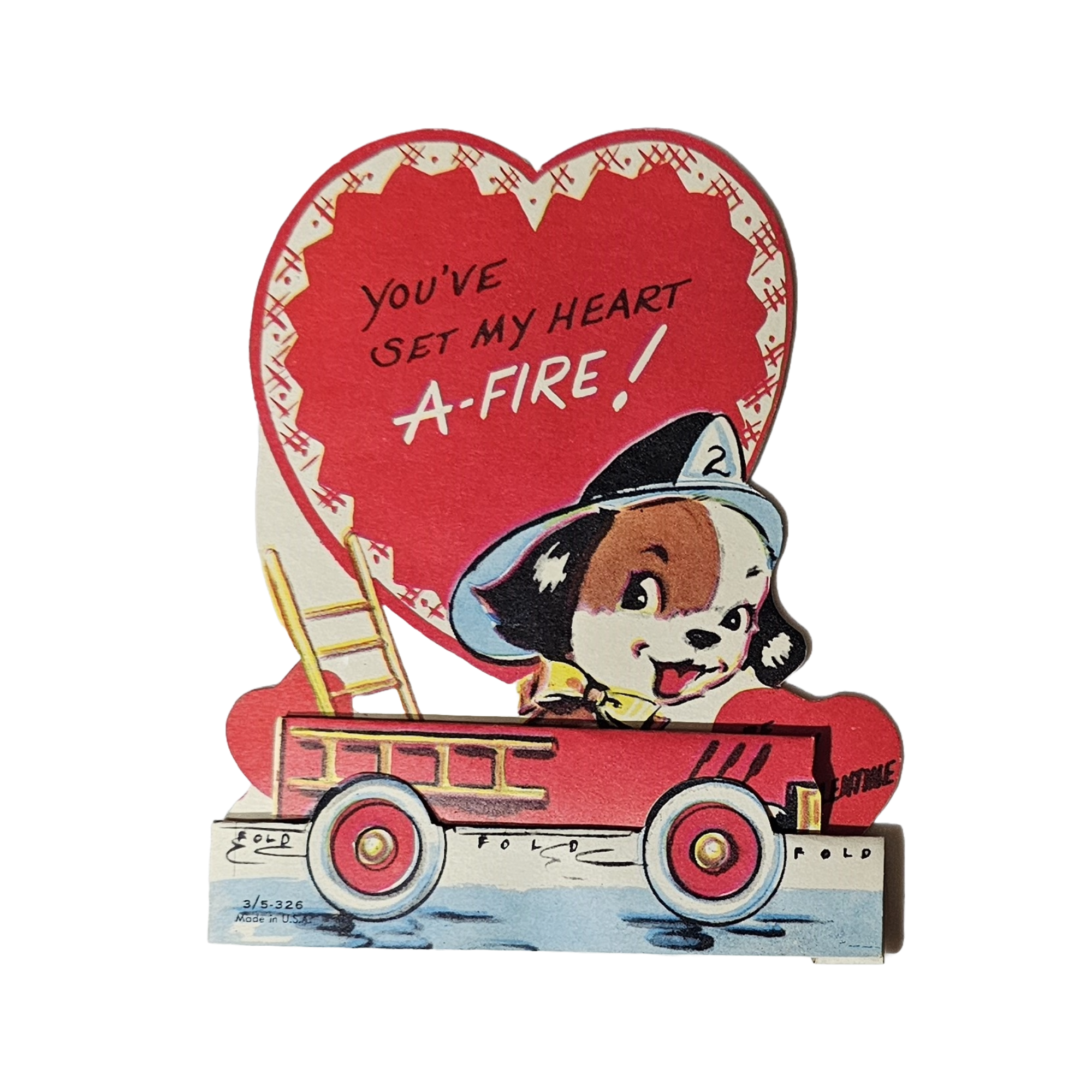The image depicts a nostalgic, hand-drawn Valentine's card set against a white background. The centerpiece is a large red heart with a white border, emblazoned with the message "You've set my heart afire!" in black and white text. Below the heart, a whimsical scene unfolds: a small fire truck with vibrant yellow ladders and white tires accented by red wheels and golden hubcaps. To the side of the fire truck, a charming brown and white dog is featured, its ears resembling human hair, adorned with a yellow bow tie and a distinctive black and white firefighter's hat marked with the number "2." In the bottom left corner, the text "35326 made in USA" is printed, and elsewhere, the word "fold" appears multiple times, suggesting it’s an old-fashioned foldable card. The overall impression is one of vintage charm, combining elements of innocence, love, and a playful fireman theme.